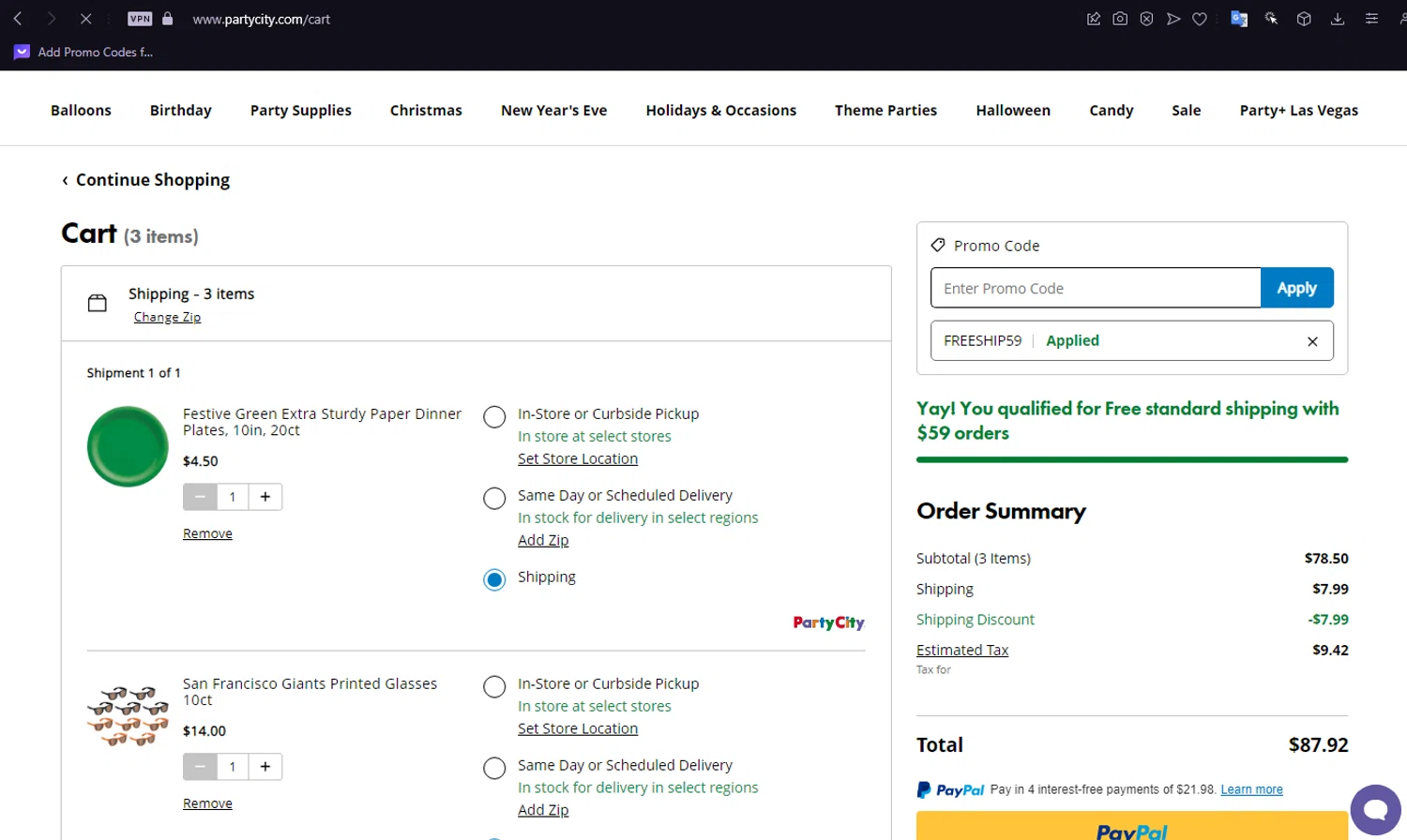Website Screenshot from PartyCity.com:

At the top of the webpage, there is a black navigation bar featuring a clickable gray back button and an X for closing. Additionally, it includes a gray VPN icon and a lock button, ensuring secure browsing on PartyCity.com. The navigation bar also displays a home icon, a camera icon, and other clickable options.

Directly below, a white menu highlights various categories available on the site: Balloons, Birthday, Party Supplies, Christmas, New Year's Eve, Holidays and Occasions, Theme Parties, Halloween, Candy, Sale, Party Star, and Las Vegas.

The main section shows the current shopping cart with three items in it. The first item listed is "Festive Green Sturdy Paper Dinner Plates," measuring 10 inches and available in a 20-count pack for $4.50. There is an option to view shipping details specific to this item, with the Party City logo displayed in multi-colors in the lower right-hand corner.

The second item is a 10-count pack of "San Francisco Giants Printed Glasses," resembling sunglasses, priced at $14 each. There are options to adjust the quantity or remove the item. However, current shipping costs for these glasses are not visible.

The details of the third item are partially off-screen and not visible in this view. Despite the seemingly mismatched choice of green plates for a San Francisco Giants-themed event, it is noteworthy that the total cart value is $87.92, qualifying for free Santa Fe shipping.